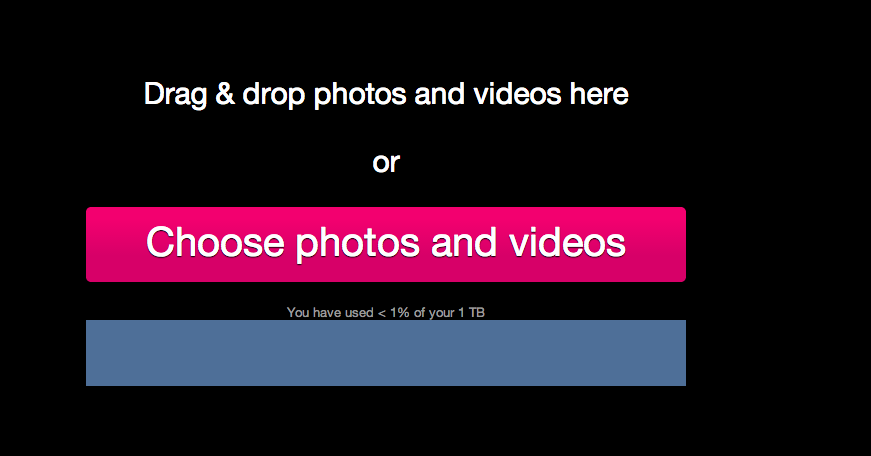The image is a graphic, likely from a website or software interface, with a solid black background. At the top, in bold white letters, it reads "Drag and drop photos and videos here." Beneath this, in smaller white text, is the word "or." Below "or," there's a prominent bright pink rectangular button with white text that says "Choose photos and videos." Toward the bottom of the image, there is a small gray text that notes, "You have used less than 1% of your 1 TB." Directly beneath this text is a muted blue rectangular bar, which seems to function as a progress or usage indicator.